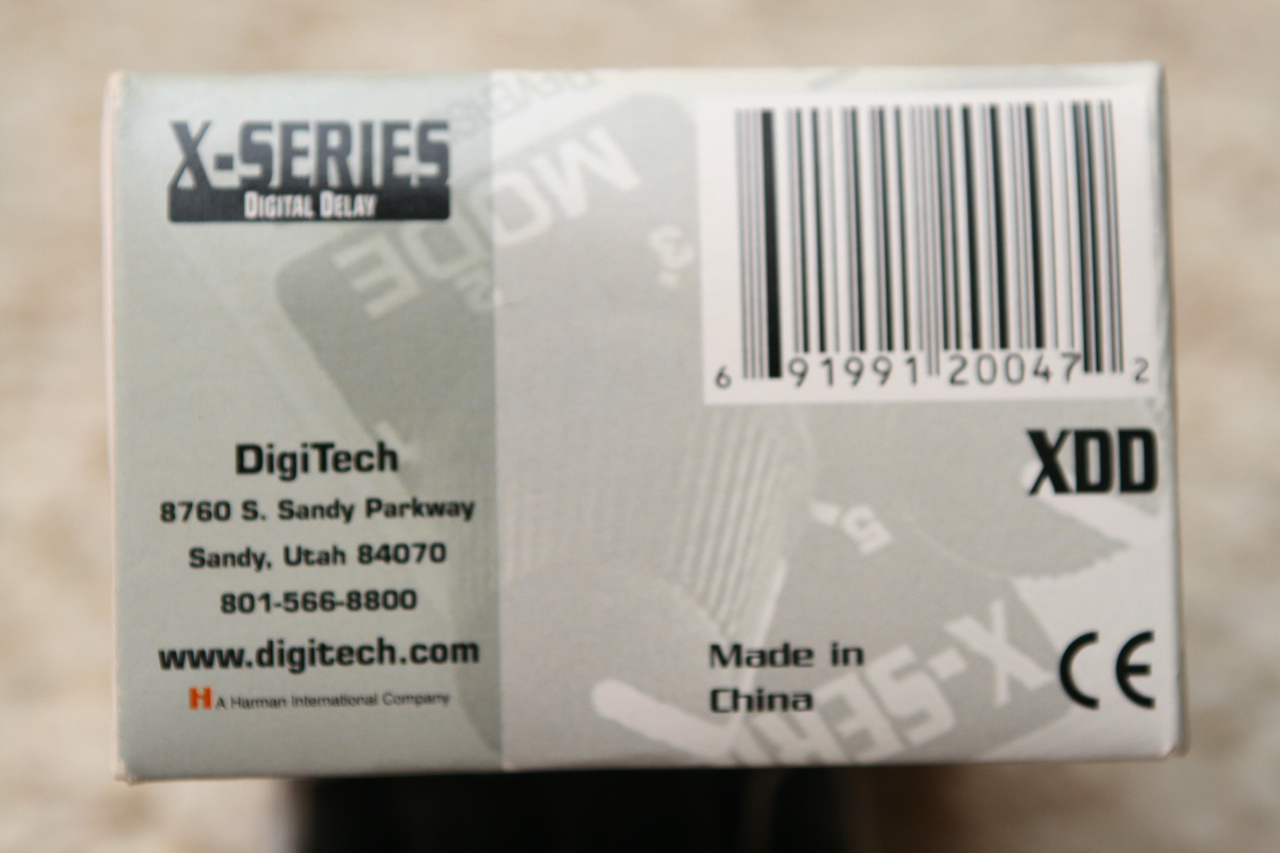This photograph captures a label with a detailed layout against a beige and cream background. The label itself is square and features a light green background. Positioned prominently in the upper left-hand corner is the text "X-SERIES" in bolded green, written in all capital letters. Directly below, a green rectangle contains the white-centered text "DIGITAL DELAY." 

A small space separates this from the next line, which reads "DIGITECH" in bolded green. Underneath, the address, phone number, and website information are printed. 

The right side of the label shifts to a whiter background. In the upper right-hand corner, a large white square displays the UPC code. Directly below the UPC code, aligned with the right edge, are the bolded black capital letters "XDD."

Centrally positioned at the bottom of the label is the text "MADE IN," followed by "CHINA" beneath it. In the lower right corner, "CE" is printed in bold black letters.